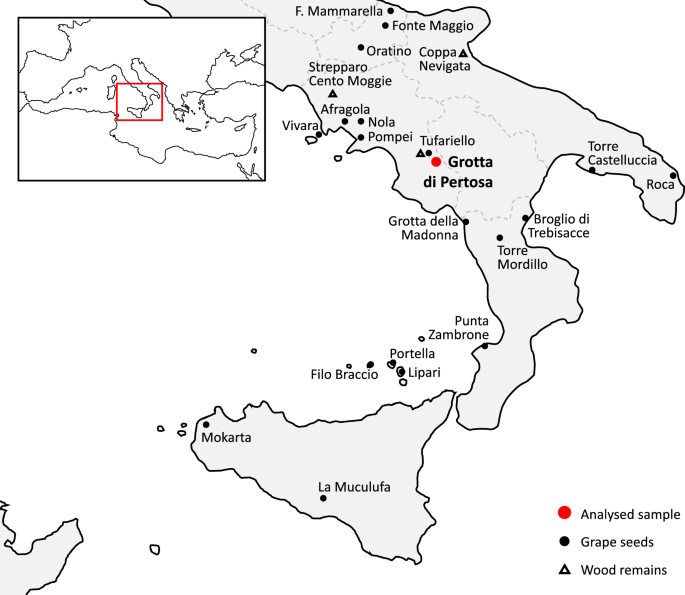This image depicts a detailed sketch of southern Italy, including the island of Sicily at the bottom left. The map prominently features large black letters at the center marking "Grotta di Pertosa," accompanied by a red dot, while other locations, identified with small black dots, include Macarta on the west side of Sicily and La Bucolufa on its bottom right. A black outlined rectangle in the upper left corner highlights the region within the broader context of Europe, with a red rectangle around the specific area depicted in the larger sketch. The map also includes a key in the bottom right corner specifying that a red dot indicates "Analyze Sample," a small black dot denotes "Grape Seeds," and a small triangle signifies "Wood Remains." Additionally, other named locations across the map are Mamarella, Fonte Maggio, Oratino, Capa, Navagata, Strapparo, Santo Maggi, Afrogola, Nola, Pompeii, Tufuriello, Torre Mordio, Rogilio di Trevisacci, Torre Castelluccia, Roca, Punta Zambroni, Portella, Lepari, Filo, Brasio, and Torre Mugello.